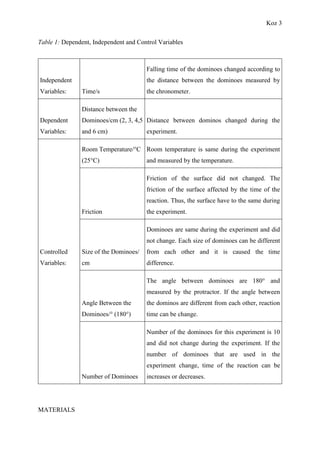Against a plain white background, there is a vertically rectangular chart divided into three main columns labeled "Dependent Variables," "Independent Variables," and "Controlled Variables." The chart features horizontal lines separating multiple sections beneath each heading. In the upper right corner, the title "Table 1" is visible. Each column contains several descriptions, though the text is very blurry and difficult to read. Key terms such as "times," "distance," "room temperature," "friction," and "angle" can be identified. The Dependent Variables section includes an explanation about the "distance between something changed during the experiment," though specific details are hard to decipher. The chart uses black text on the white background, and there's an additional note about "Materials" in the bottom left corner. The text generally remains small and blurry, making it challenging to read the finer details.